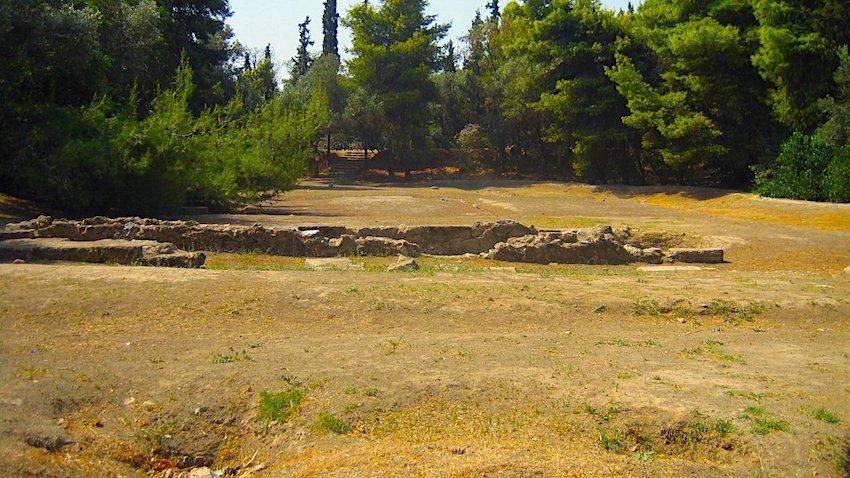The photograph, taken outdoors on a sunny day, is a square, full-color image of a serene field framed by a clear blue sky and a dense line of lush coniferous trees at the top. The landscape is composed of an open expanse of dirt and patches of grass, which appear somewhat yellowish and dead in some areas, indicating a dry season. Dominating the center of the image is the remnants of an ancient, dilapidated rock wall. The wall, composed of short, brown stones that barely reach knee height, is broken and incomplete, suggesting the passage of time. The rocky structure runs horizontally across the center and blends into the aged field, creating a stark contrast against the vibrant treeline and the clear, open sky above. There are no people, animals, or text in the photograph, allowing the viewer to fully take in the natural and historical elements of the scene.